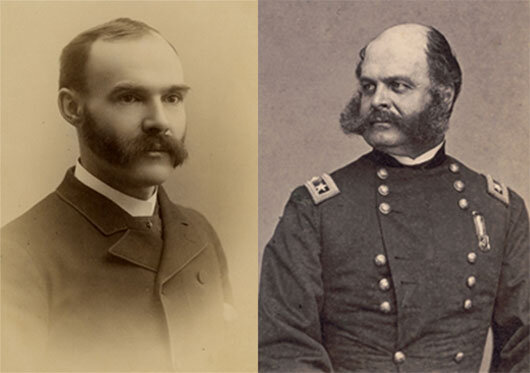The image comprises two side-by-side grayscale photographs, each displaying a man from a bygone era, suggesting a historical context likely related to the military. The left photograph exhibits a man with a distinct mustache that seamlessly blends into his sideburns while leaving his chin clean-shaven. He has a receding hairline and wears a button-up jacket with a white collar underneath. The background appears to be a light tan or cream color, evoking an aged and timeless feel. This man gazes diagonally to the right.

The right photograph showcases an older man who bears a striking resemblance to the one on the left, hinting that they might be the same individual at different stages of life. His hairstyle similarly includes balding on top with hair along the sides, and he sports a fuller, more unkempt version of the mustache-sideburn combination. He is adorned in an elaborate military uniform featuring numerous buttons arranged symmetrically along the torso and patches with stars on his shoulders. This man looks to the left, and the background is a muted gray, adding to the vintage atmosphere of the portrait. The clean, empty backgrounds in both photographs highlight the men's detailed features and uniforms, emphasizing their potential historical significance.